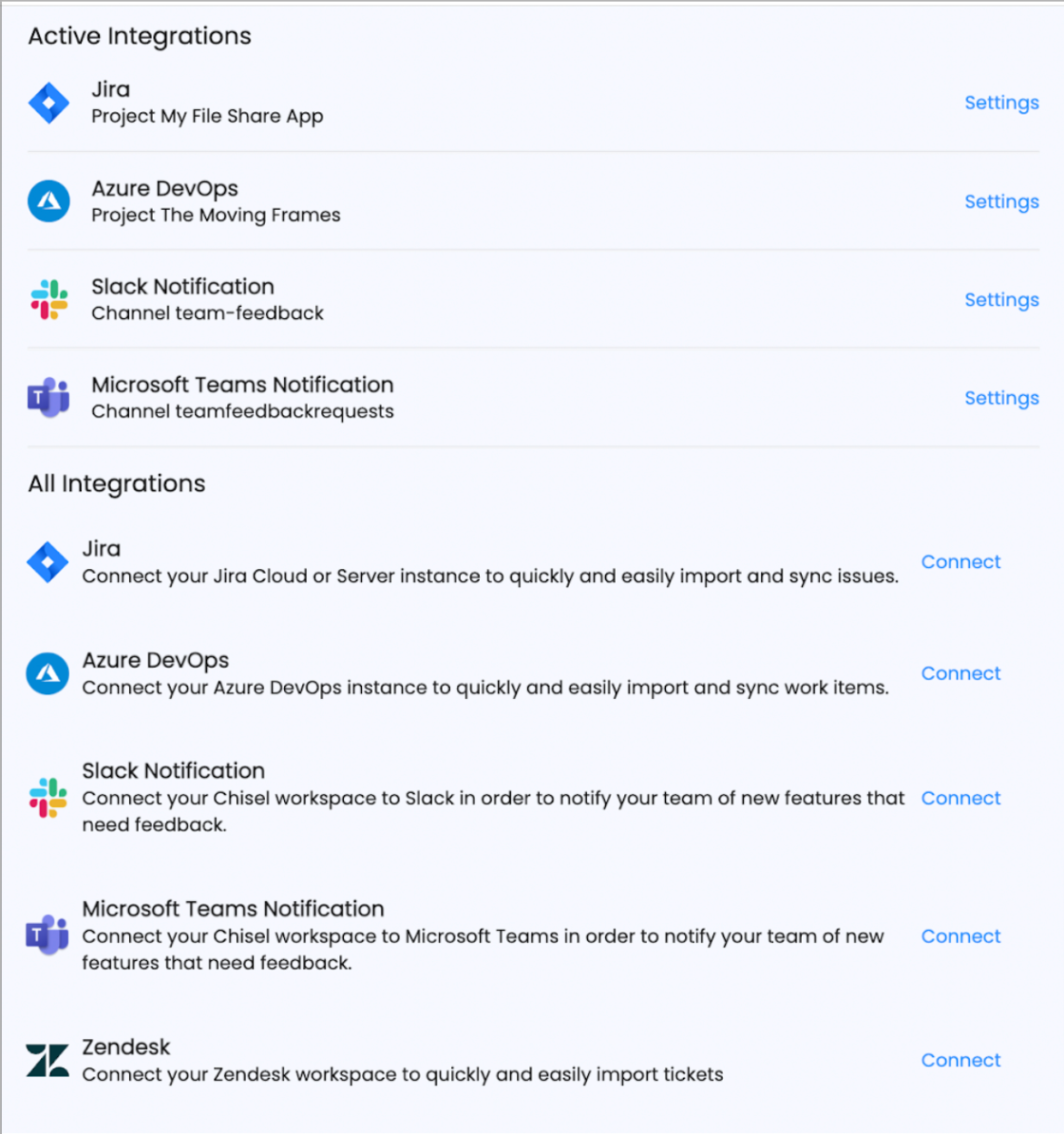The image depicts a webpage with a clean, white background and primarily dark or black text. At the top of the page, a header reads "Active Integrations." Below this header, various columns and options are listed in a top-down format.

1. **JIRA Protect My File Share App**: This appears as the first item.
2. **Azure DevOps Project: The Moving Frames**: Listed as the second option.
3. **Slack Notification Channel: Team Feedback**: The third item.
4. **Microsoft Teams Notification Channel: Team Feedback Request**: The fourth item.
5. **All Integrations**: This is another section heading.

Continuing further down the page, each integration is accompanied by a brief description detailing its functionality:

- **JIRA**: "Connect your JIRA Cloud or Server instance to quickly and easily import and sync issues."
- **Azure DevOps**: "Connect your Azure DevOps instance to quickly and easily import and sync work items."
- **Slack Notification**: "Connect your Chisel workspace to Slack in order to notify your team of new features that need feedback."
- **Microsoft Teams Notification**: "Connect your Chisel workspace to Microsoft Teams in order to notify your team of new features that need feedback."
- **Zendesk**: "Connect your Zendesk workspace and easily import tickets."

The webpage seems to be a dashboard where users can manage and configure various integrations with different productivity and collaboration tools, facilitating seamless workflow and communication across platforms.